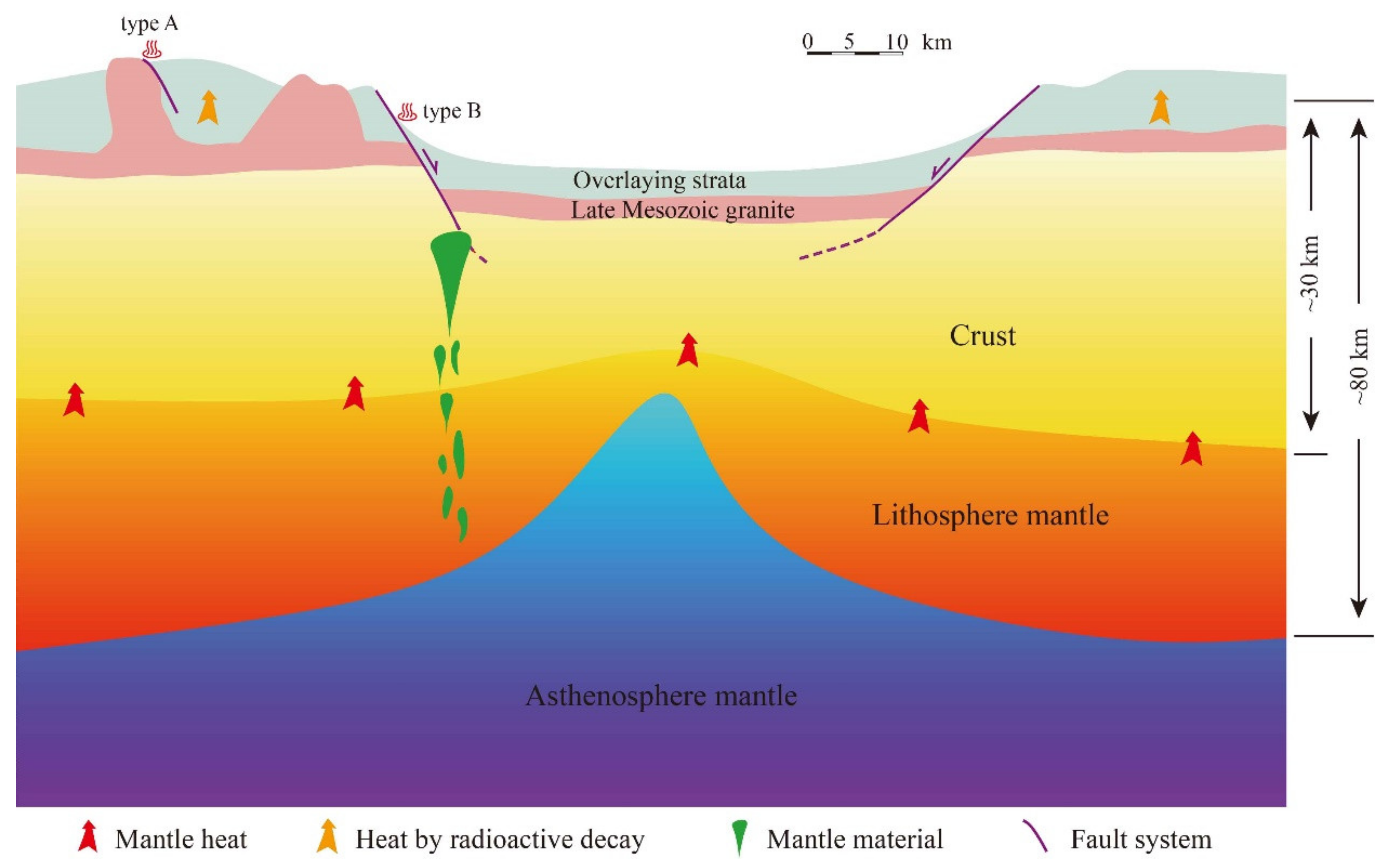The illustration is a detailed geological diagram depicting the various layers of the Earth's crust. At the top, it begins with a water layer, followed by the overlaying strata depicted in light gray. Above the crust, the late Mesozoic granite is represented in pink, with parts protruding above the water. The Earth's crust is shown in a yellow shade, beneath which lies the lithosphere mantle colored orange. At the bottom, the asthenosphere mantle is colored blue. The diagram includes several scale markers and labels, with one side displaying distance markers such as 30 kilometers and 80 kilometers, and the top featuring a ruler to help gauge the separation between different layers. Additionally, there are various annotations and arrows indicating forces at play, including a red arrow for mantle heat, a yellow arrow for heat by radioactive decay, a green arrow for mantle material, and a diagonal purple line denoting the fault system. The bottom of the diagram also includes detailed text specifying terms like the mantle, fault systems, and heat dynamics, providing a comprehensive view of the subsurface geological structures.